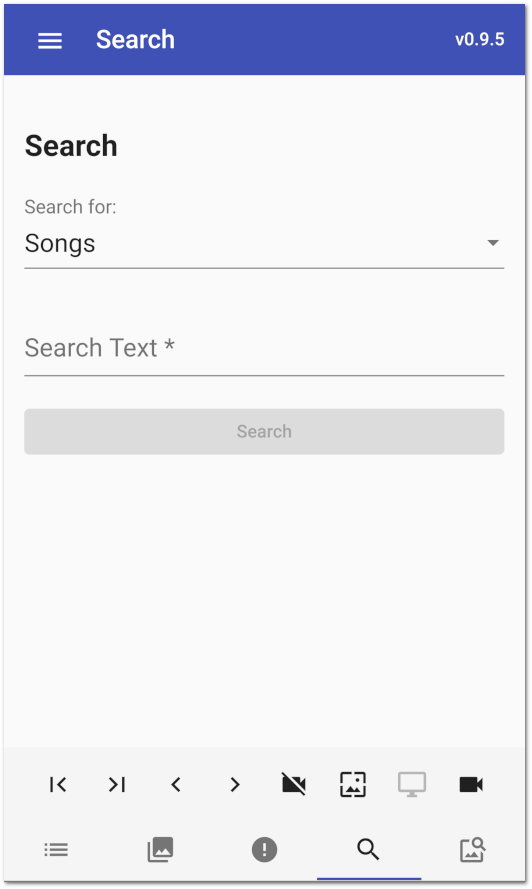The image depicts a device screen with a blue top bar extending across the width. On the top left of this bar is a "More" icon, followed by a "Search" option. The top right corner displays the version number "V0.9.5". Below the blue bar, the screen has a white background section. On the left of this section, the word "Search" appears, followed by the text "search for:" beneath it. Further down is a tab labeled "Songs", with a black downward-pointing arrow on the far right. The text "Search text *" is situated below this tab. A gray button with the word "Search" in the middle is also included below this text field. At the bottom of the screen, there are two rows of icons. The top row consists of a "Back Pause" button on the far left, a "Forward Pause" button to its right, followed by a standard "Back" button, and then a "Forward" button. The rightmost icon on this row is an image of a crossed-out camera.